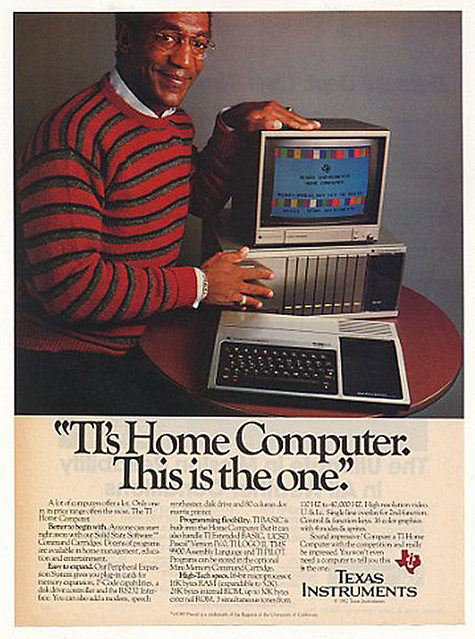This image is a vintage advertisement from the early 1980s for Texas Instruments. It features a younger Bill Cosby, the renowned American actor and comedian. Cosby, a black man, is seen smiling at the camera while slightly reaching out over an old-school computer, reminiscent of the 80s. He is dressed in a red, gray, and black striped sweater with a white collared shirt underneath, the collar peeking out over the sweater. He also wears oval-shaped glasses. The main text reads, "TI's Home Computer. This is the one." although much of the subsequent text is blurred due to the age of the ad. The Texas Instruments logo, a red depiction of the state of Texas with a "T" and a white "I," is prominently displayed in the bottom right corner of the image.